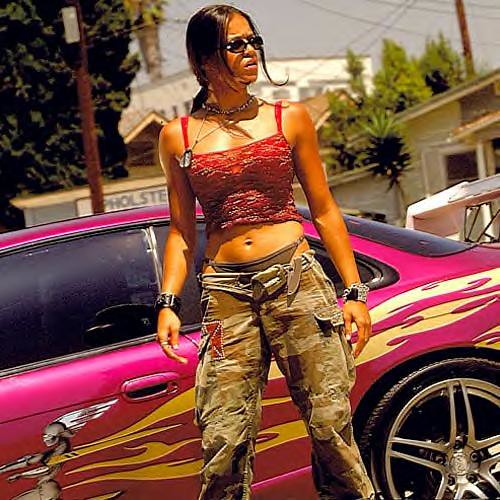The image features actress Michelle Rodriguez, portraying her character from the movie "Fast and Furious." She stands confidently in front of a flashy, bright pink sports car adorned with beige and white decals resembling wings or flames. The car sports shiny silver chrome wheels, tinted black windows, and is parked on an urban street. Michelle has short dark brown hair pulled back into a ponytail with heavy wisps framing her face, and her expression appears somewhat concerned as she gazes off to the right.

Michelle is dressed in a fashionable urban outfit comprising a red spaghetti-strap tank top that reveals her midriff, brown thong underwear partially visible above her camouflage cargo pants, which are unbuttoned and ride low on her hips. Around her neck, she wears dog tags, and on her wrists are heavy metal bracelets. Her stance is assertive, with her feet planted far apart and her elbows slightly bent.

In the background, the surroundings include an upholstery store or shop, several houses, a tall white building with gray trim, and various tall green palm trees. There are visible elements like a red pole, a brown light pole, and power lines. The sky above is clear and blue, indicating a sunny day.